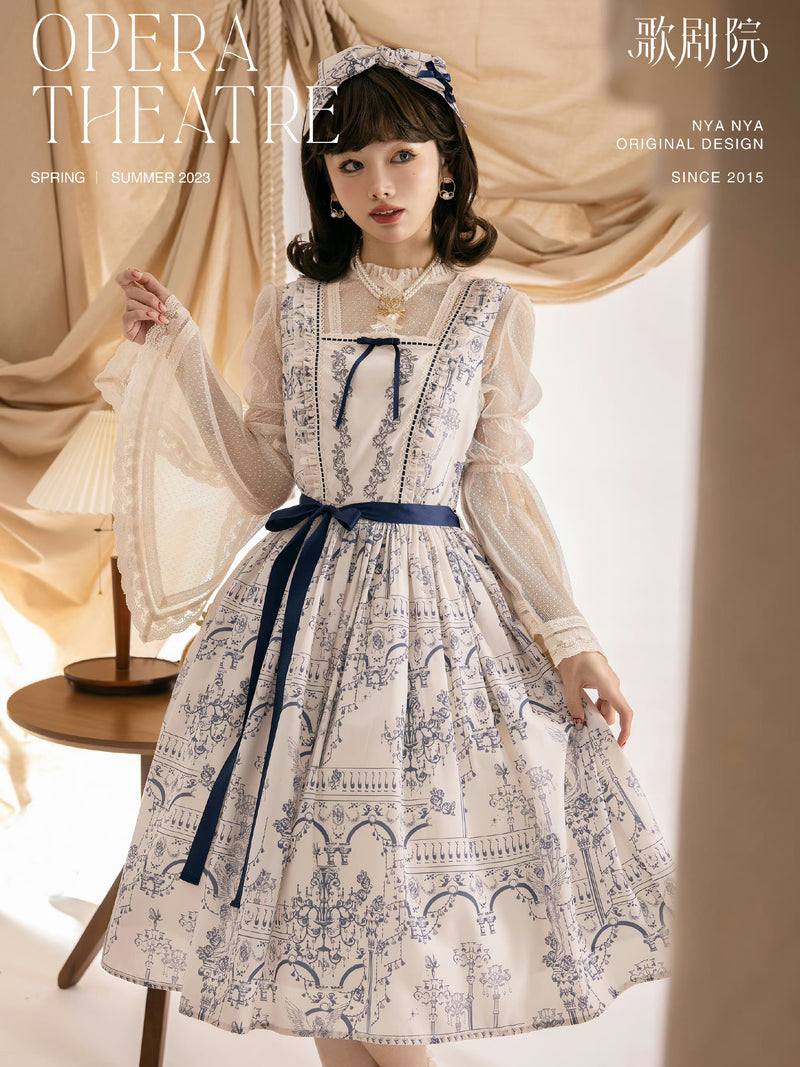The image depicts a magazine cover titled "Opera Theatre," showcasing its Spring and Summer 2023 edition. Dominating the cover is a young Asian woman, elegantly dressed in a Victorian-style white dress adorned with blue ribbons and intricate lace sleeves. Her hair is styled in old-fashioned curls with bangs framing her face. The dress features a dainty blue design of a cityscape with floral intricacies, possibly depicting a Renaissance-era French bridge. To the left side of the cover, the magazine title is displayed, while the right side features three Asian characters and the phrase, "N.Y.A. N.Y.A. original design since 2015." The model's pose suggests motion, with her right arm raised and her left hand holding her skirt as if preparing to bow. In the background, a cozy living room setting is visible, including a brown table topped with a lamp featuring a brown base.